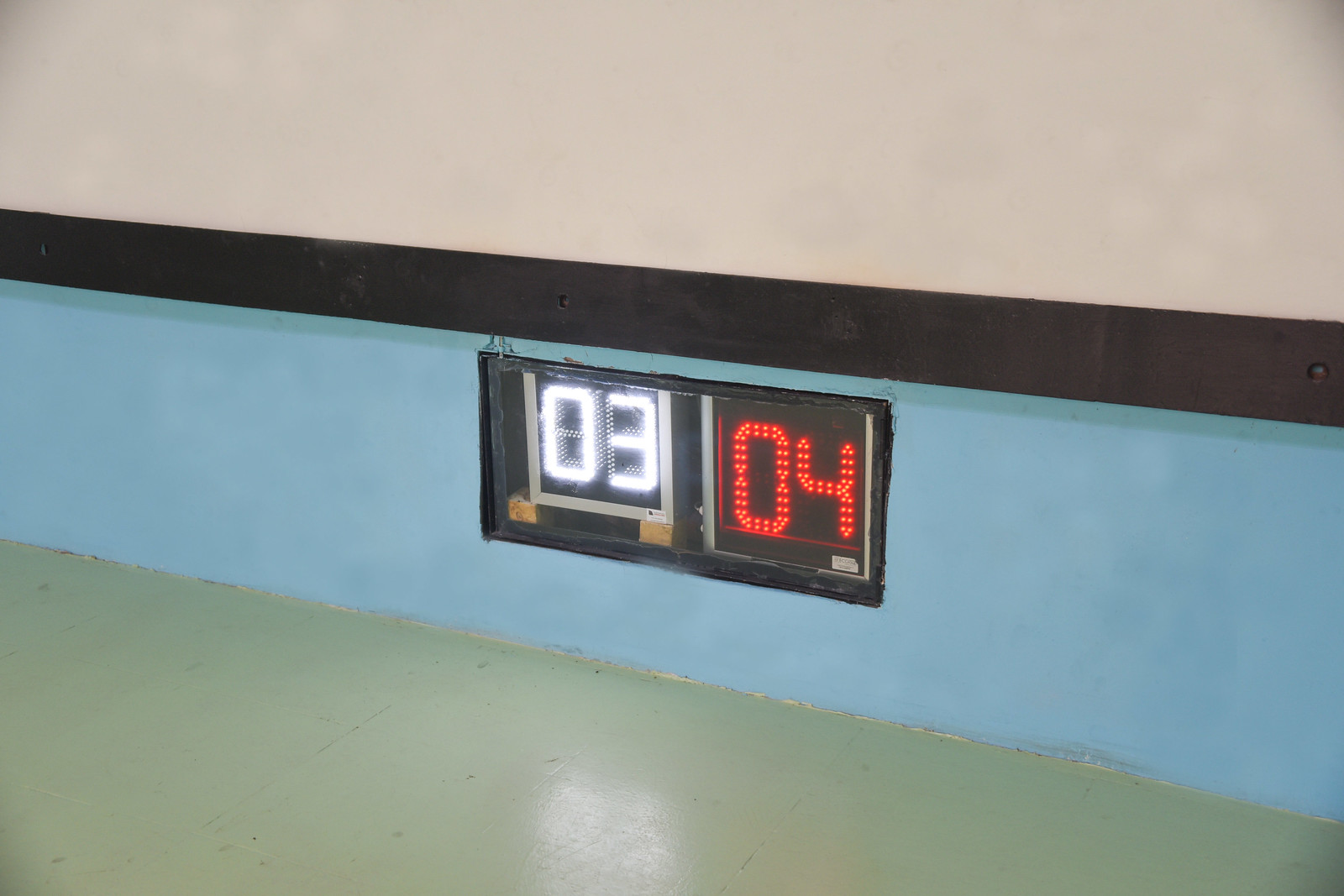The image shows a misaligned digital scoreboard embedded into a section of a gym or indoor recreational wall, possibly close to the floor area. The floor beneath the scoreboard is painted gray, resembling concrete. The base of the wall, where the scoreboard is set into a cutout, is blue. Above this blue section, there is a flat black railing against the wall, and the upper portion of the wall is whitish in color. The cutout contains two different digital display boxes: the smaller left one with white numbers displaying "03," and the larger right one with red numbers displaying "04." The left display is noticeably propped up by wooden blocks and is misaligned compared to the flush-mounted right display.